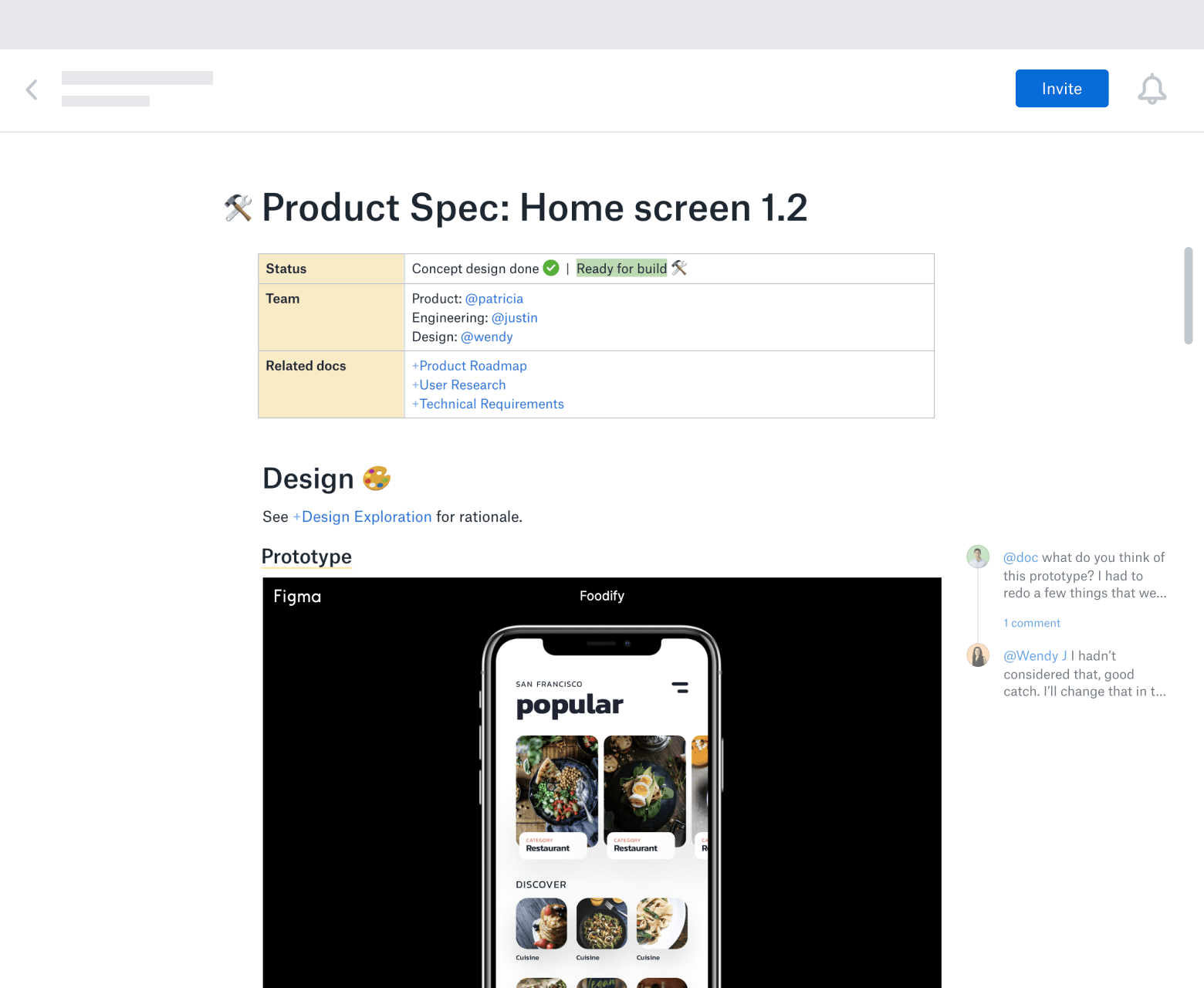A snapshot taken from a smartphone showcases a comprehensive project management screen titled "Product Spec: Home Screen 1.2." The screen features a status chart displaying "Concept Design" with a checked mark indicating completion, and "Ready for Build," accompanied by tool icons. The team section highlights responsible members: Product (@Patricia), Engineering (@Justin), and Design (@Wendy). 

On the left, a section labeled "Related Docs" lists essential documents such as the product roadmap, user research, and technical requirements. Below, the design area is marked by an artist's palette icon, suggesting ongoing creative efforts. 

An embedded prototype display within a black rectangle illustrates a mobile app interface created in Figma for a project named "Foodify" based in San Francisco. The app's home screen shows popular food dishes with a "Discover" section, presenting various cuisines and restaurant recommendations.